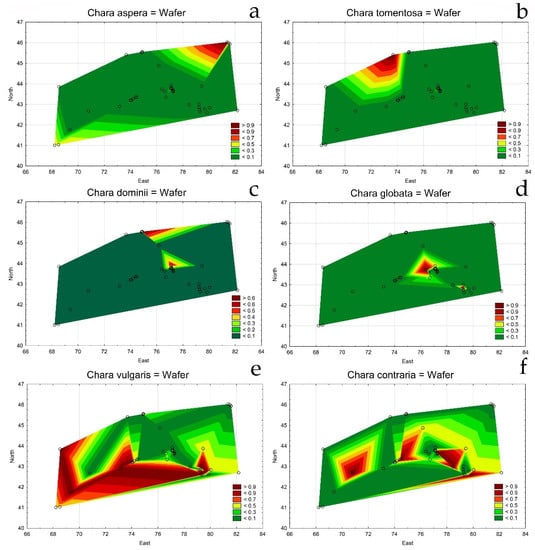The image is a detailed grid of six graphs, each labeled from A to F, arranged in a two-by-three collage. Each graph depicts a rectangular area covered with various colors, indicating different intensity levels. The labels in a different language read as follows: A - Chara Aspera = wafer, B - Chara Tementosa = wafer, C - Chara Domini = wafer, D - Chara Globata = wafer, E - Chara Vulgaris = wafer, and F - Chara Contraria = wafer. Along the left side of each graph is a vertical axis labeled "North" with incremental values from 40 to 47, and along the bottom, a horizontal axis labeled "East" stretching from 66 to 84, increasing by twos. The graphs prominently feature a gradient of colors, ranging from dark red to dark green, represented in a legend situated at the bottom right of each chart. Despite some uncertainty about the specific data, the coloration is likely indicating varying levels, possibly related to weather, heat, or some form of intensity measurement.